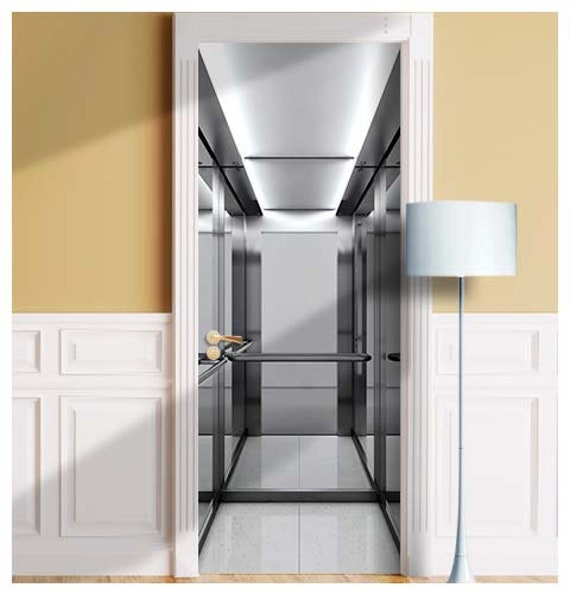The image depicts a hallway, potentially in an apartment complex, leading into a separate, more sterile-looking room. The initial room features light brown or tan walls with white paneling along the lower half and a tall, thin white lamp with a shaded top to the right. The hallway ahead has glass flooring and mirrored walls on either side, creating a reflective, metallic appearance that lends a sense of spaciousness and modernity. This glassy corridor is well-lit from above by out-of-focus ceiling lights that cast a subtle glow. The far end of the hallway transitions into another glass-walled corridor that appears to arch left and right, further enhancing the sense of depth and multiple directions within the space.